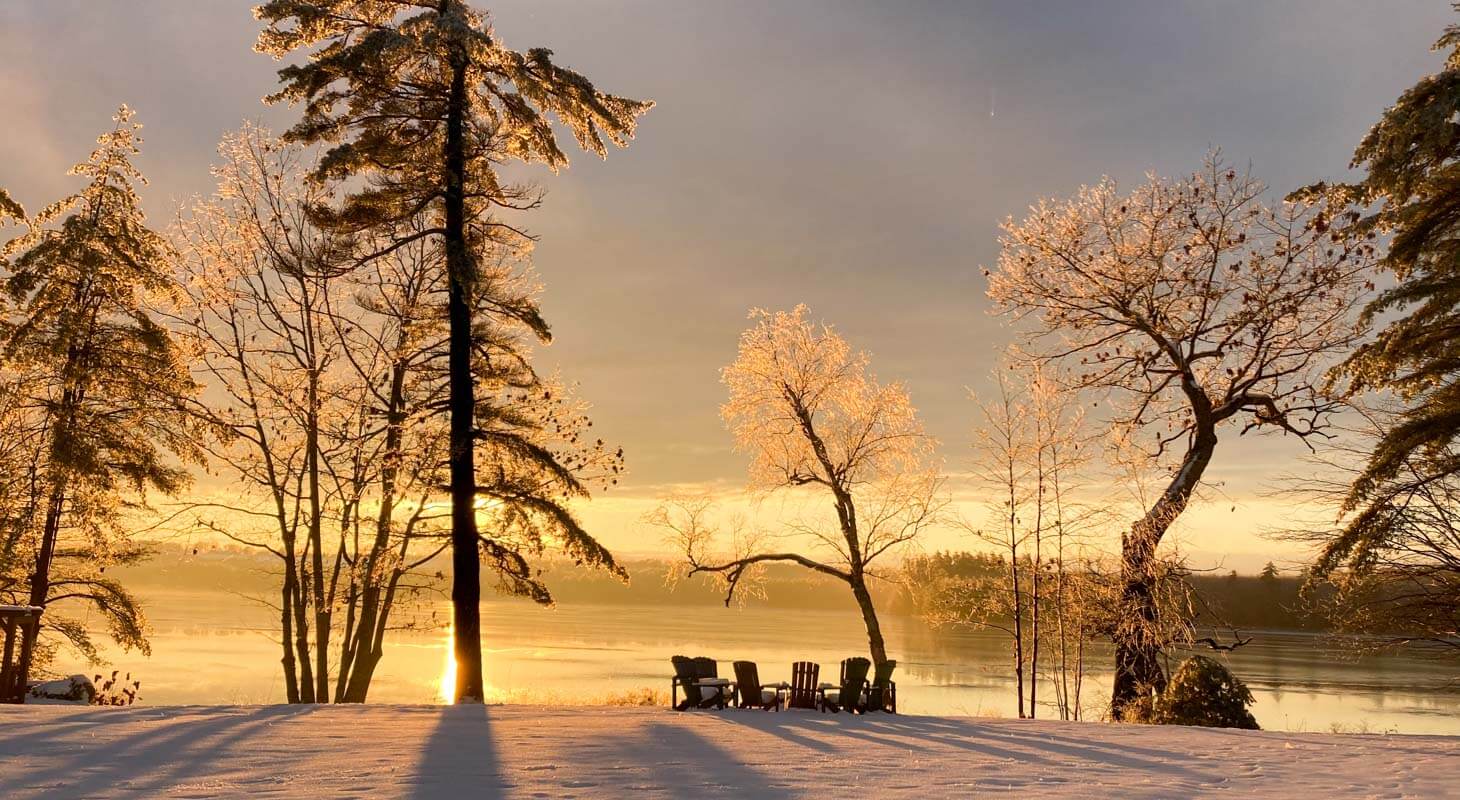This is a horizontal outdoor photograph capturing a serene, winter sunset scene by a large lake. The ground in the foreground is blanketed with snow and ice. There are six wooden lounge chairs arranged in a semicircle, possibly around a campfire site, though no fire is visible. Tall, thin trees, some evergreen and others leafless, frame the scene, casting long, angled shadows on the snowy ground. The still, flat lake, which spans the entire width of the photo, mirrors the golden light of the setting sun, peeking through the trees on the middle left side. The sky transitions from a bright yellow near the horizon to darker blues and grays higher up, creating a striking contrast with the sepia-toned landscape. In the distance, mountains are faintly visible through the gaps in the trees, adding depth and context to this tranquil, nature-filled moment.